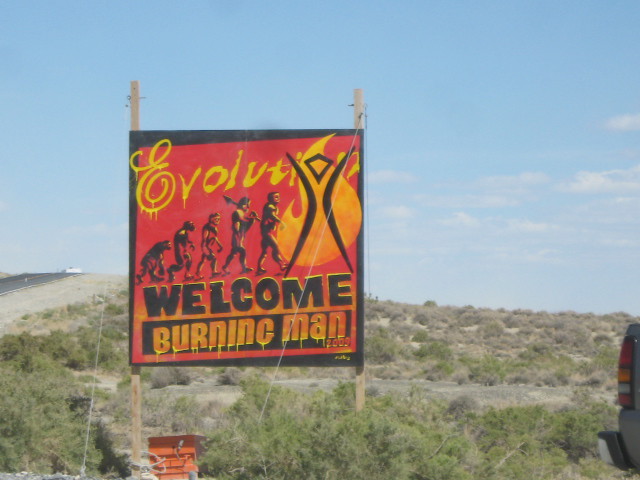In this captivating desert scene, a pristine blue sky adorned with fluffy white clouds stretches above an arid landscape. A rugged dirt and gravel road meanders through the setting, leading to a small hill crowned by a white vehicle. To the side of the road, a lone black object punctuates the terrain, surrounded by a scattering of green and brown shrubs.

Dominating the scene, a massive red dump truck stands alongside another truck parked nearby. The focal point, however, is a striking sign mounted on two wooden posts. This sign features a bold red background accented with black borders. Prominently displayed in yellow letters, the word "EVOLUTION" arcs above a sequence of images depicting the progression from monkey to modern man. The word "WELCOME" is inscribed below in black. Another prominent feature of the sign is a black square with "BURNING MAN" written in yellow, completing this vivid and thought-provoking tableau.